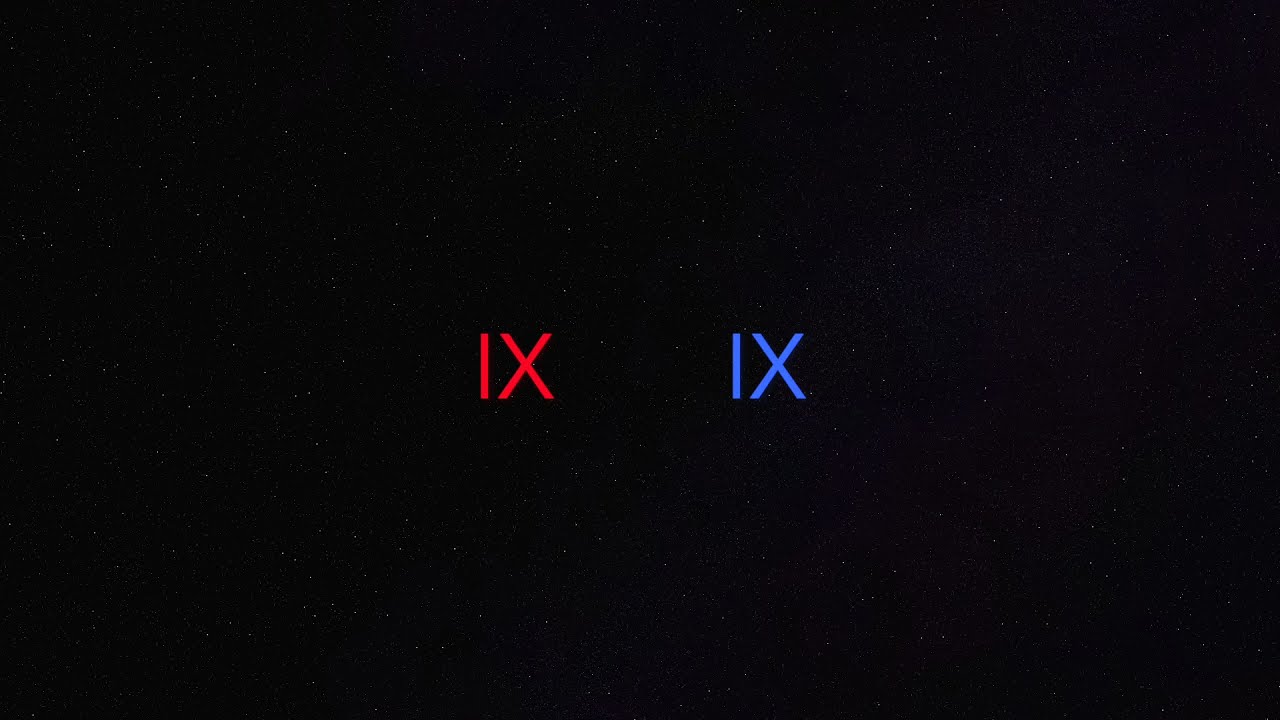This digital image, set against a black background that mimics a starry night sky, is rectangular in landscape orientation. The black background is peppered with numerous tiny white flecks and some off-white, light yellow, and faint blue specks, resembling distant stars. In the center of the image, both horizontally and vertically, are two sets of uppercase Roman numeral IXs. The IX on the left is red, while the IX on the right is blue, each with about a half-inch of space between them. These Roman numerals are centrally justified, ensuring a balanced appearance against the celestial backdrop. The overall effect is a minimalistic yet striking representation of a night sky with vivid red and blue Roman numerals prominently displayed in the middle, surrounded by a universe of tiny stars.